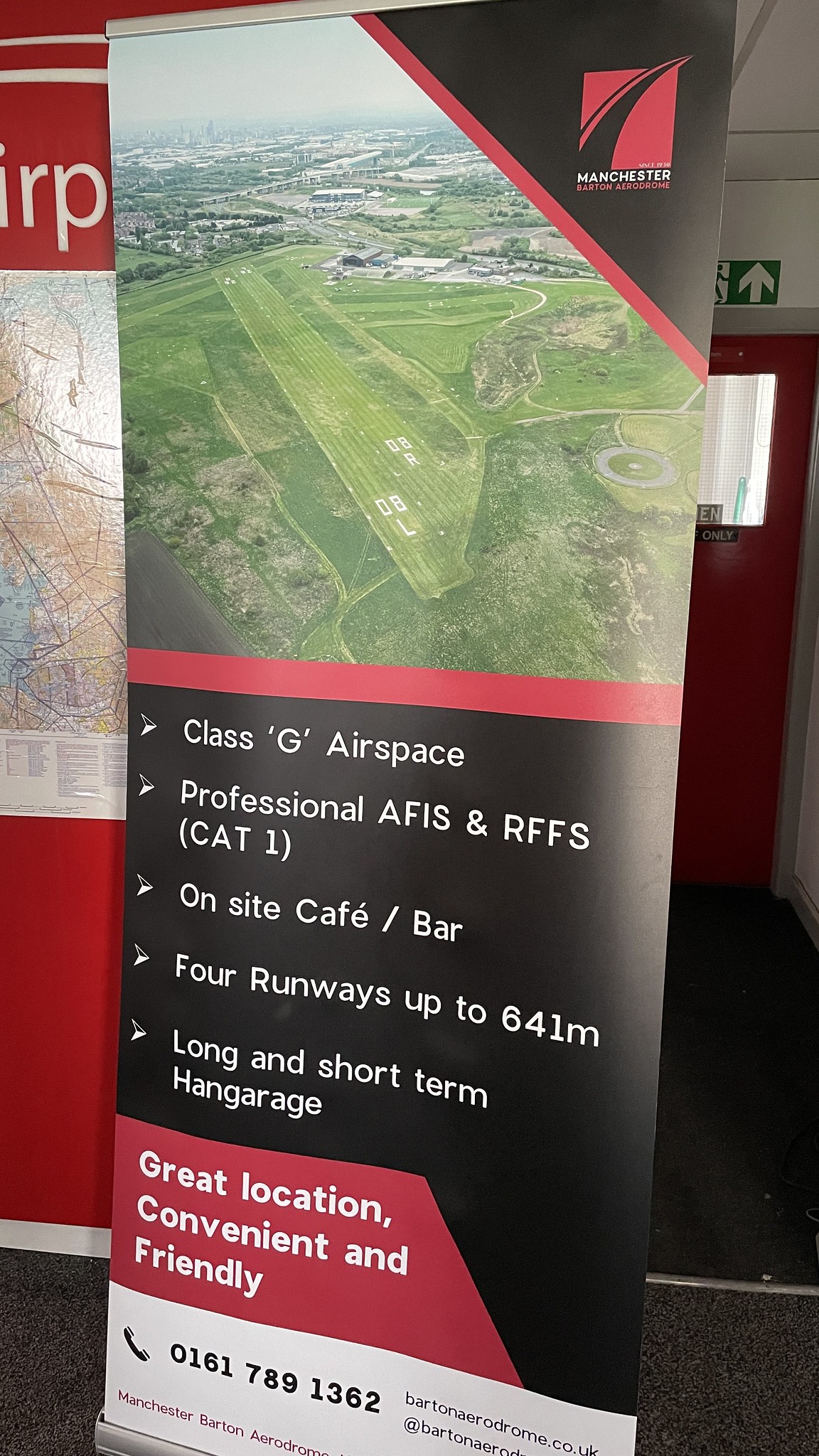This image features a promotional banner for Manchester Airport, likely displayed indoors at an event or a trade show. The banner, predominantly black with red stripes and white text, showcases a detailed aerial photograph of the airport, presenting a green field with vast grassy areas and a distant cityscape. The top right corner of the banner bears the Manchester logo in red. Below the photograph, the text describes the airport's features: "Class G airspace, professional AFIS and RFFS, Cat 1, on-site café/bar, four runways up to 641 meters, long- and short-term hangarage." Additionally, it highlights benefits with phrases in red such as "great location, convenient, and flight-friendly." The fine print at the bottom includes contact details like an email address and the phone number 0161-789-1362. The detailed layout emphasizes the airport's amenities and strategic advantages for potential users.